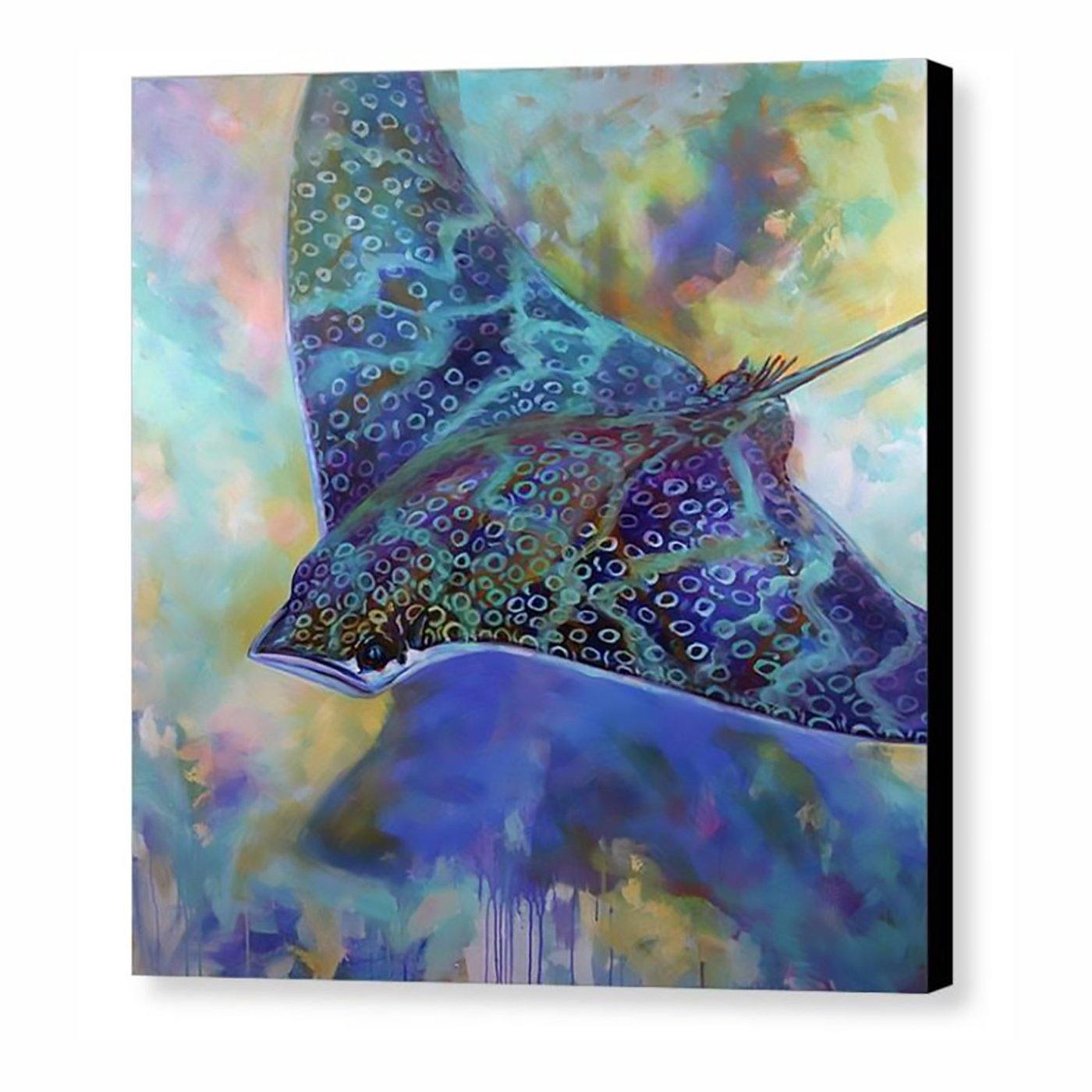This painting features a vividly colorful depiction of a stingray, with its dynamic form being the focal point of the artwork. The stingray is detailed with a predominantly dark blue body adorned with swirling, fluorescent green patterns and distinct white circular markings. Its eyes are blue, and it has highlights of yellow and white stripes that add depth and contrast to its features, including a white underbelly and mouth, and a stinger prominently visible at the back.

The background, while not resembling a typical ocean scene, enhances the surreal quality of the painting. It's composed of a mix of bright, vibrant hues—pinks, purples, blues, greens, yellows—blended in a watercolor style that gives a psychedelic effect. These colors merge into a kaleidoscopic array that makes the stingray appear as though it is swimming through an otherworldly, dream-like space, further emphasized by the blue splotch at the bottom that anchors the composition. The entire piece rests on a white canvas, making the explosion of colors even more striking against the neutral background behind the painting.